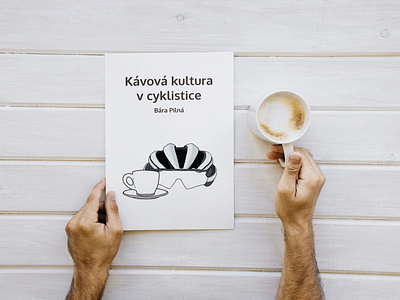In this aerial shot, we see the forearms and hands of a man holding a sign and a coffee mug against a white wooden surface composed of six horizontal slats. The man's right hand, characterized by dark hair and some visible arm hair, grips a white coffee mug, which has a light brown residue inside, hinting at prior consumption. His left hand, showing the top knuckles and thumb, holds a white piece of paper. The paper displays text in a foreign language, possibly Polish, reading "Kavova Kultura Vcyklistice," accompanied by a drawing of a helmet with a visor and a coffee cup on a saucer. This detailed composition indicates a casual moment, centered on coffee culture with a potential cyclist theme.